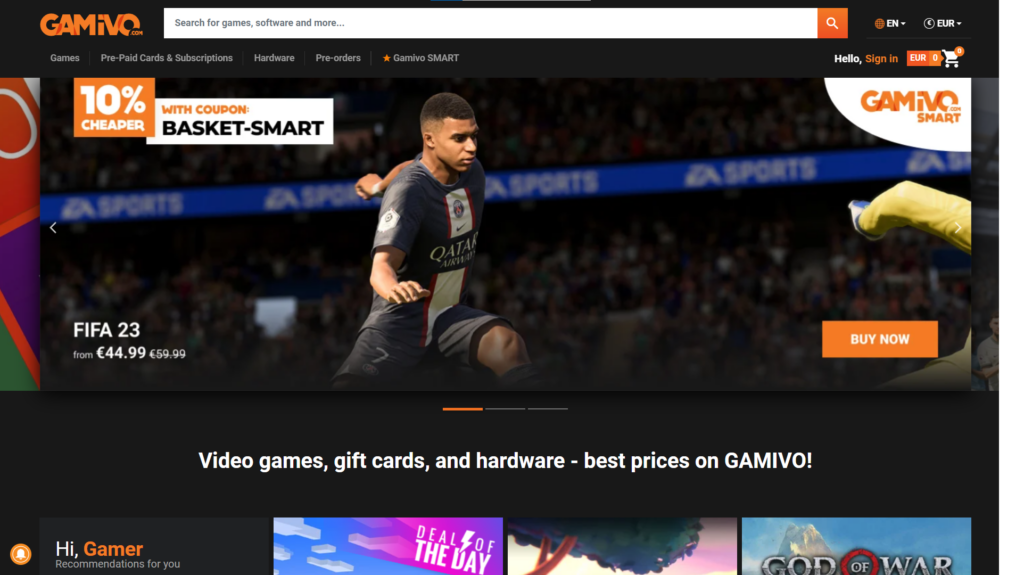A cropped screenshot of the Game Evo website's main page with a sleek black background. The top left features the Game Evo logo, while a prominent search bar sits to its right, displaying the placeholder text "search for game software and more" in small grey letters. On the far right, language preferences can be adjusted via a drop-down box labeled "English," and currency settings, currently set to Euros, can be changed using an adjacent drop-down menu.

Directly below this, a large, captivating image showcases FIFA 23 gameplay. In the bottom right corner of the image, "FIFA 23" is displayed along with pricing information: "from $44.99," where $59.99 is crossed out in small grey letters to indicate a discount. An orange "Buy Now" button is prominently positioned below the pricing.

Centered beneath the game image are three horizontal small lines. The first is colored orange, and the other two are grey, indicating FIFA 23 as the first item in a photo carousel. Below this are the words "Video games, gift cards, and hardware. Best prices on Game Evo."

The bottom right of the screen greets users with "Hi Gamer," and to the right are the partial thumbnails of three other game titles, suggesting more deals or featured items that are cropped out of the view.